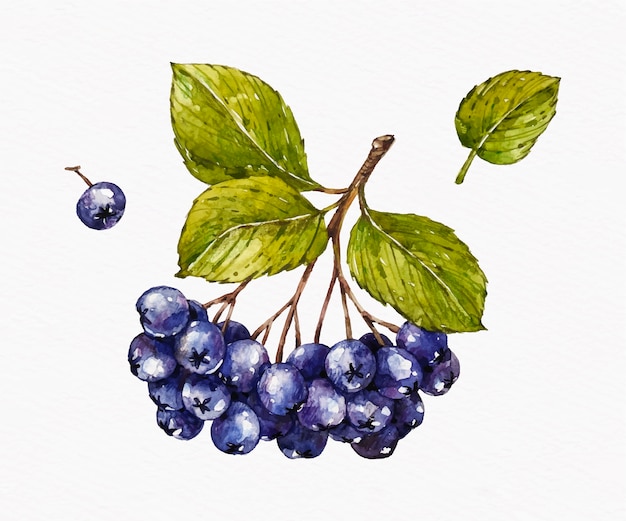This detailed illustration, rendered in a watercolor or print botanical style on white parchment-like paper, showcases a large, vivid cluster of blueberries attached to thin brown twigs stemming from a broken branch. The densely packed blueberries exhibit a gradient of blue to purple hues, each adorned with the classic star-shaped blossom end. A trio of large green leaves is prominently displayed on the severed branch, enhancing the cluster’s natural beauty. To the upper left of the composition, a single blueberry is depicted in isolation, while a solitary green leaf occupies the upper right corner, adding to the composition's balance and charm. The overall presentation captures the delicate artistry of the blueberries with a soft, bleed-y color effect, evoking a watercolor's gentle touch.